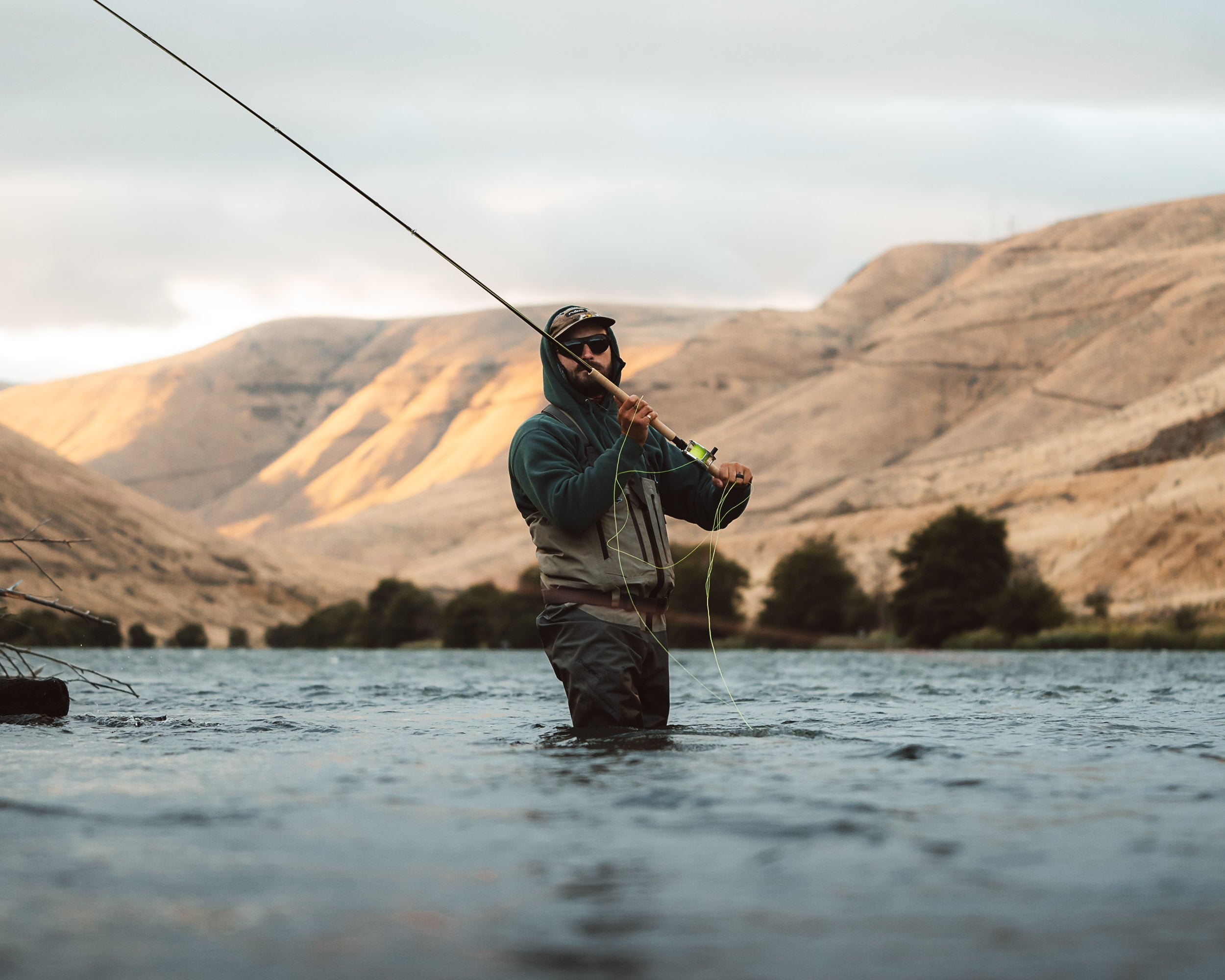The digital photograph captures a man fishing in a serene lake, with waist-deep, cold water that comes up past his knees. The man stands steadfastly in the water, dressed unusually for the activity in black jeans and a distinctive hoodie—forest green on top and gray on the bottom. He wears black sunglasses and a baseball cap under his hoodie, enhancing his focused demeanor. His fishing pole, held firmly with both hands and cocked back over his right shoulder, suggests he is just about to cast his line. Surrounding him is a picturesque backdrop of brown mountains and scattered clouds drifting across a grayish sky. The scene hints at late fall or winter, with the colors primarily brown and blue, accented by touches of light and dark green from distant trees and other elements in the landscape. Notably, there are no boats or close land in sight, adding an intriguing element to how he reached such a deep part of the lake.